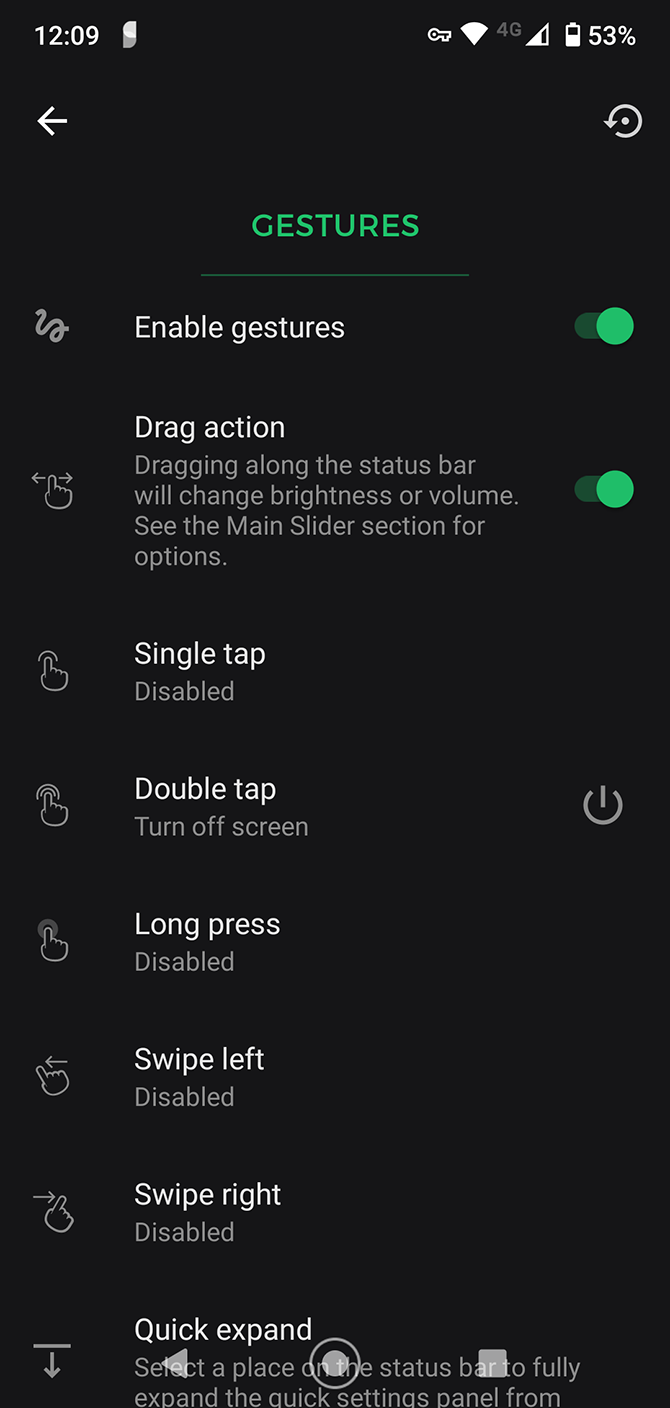A detailed and meticulously organized description of the cell phone screen image follows:

The image showcases a cell phone screen with a black background and white font. At the top of the screen is the status bar, which displays the following elements from left to right: the time "12:09," an icon representing a key, a data connection symbol indicating "4G," signal bars for the phone's connectivity, and a battery icon showing 53% charge.

Directly beneath this status bar, on the left side, there is a left-facing arrow icon. On the right side of this section, there is a button labeled "Research."

Moving down to the next section, centrally located, the word "Gestures" is prominently displayed in green, underscored by a green line. Below this heading, the text "Enable Gestures" appears, accompanied by a green toggle switch indicating that this feature is turned on.

Further details are provided under the "Drag Action" heading, which explains that dragging along the status bar will either change the brightness or volume. Users are instructed to refer to the main slider section for more options, and this feature is toggled on as well.

Below "Drag Action," there are settings for different gestures:
- "Single Tap" is disabled.
- "Double Tap" turns off the screen, with a power button icon to the right.
- "Long Press" is disabled.
- "Swipe Left" is disabled.
- "Swipe Right" is disabled.

Lastly, a partially visible section labeled "Quick Expand" describes selecting a spot on the status bar to fully expand the quick settings panel, but the description is cut off and incomplete.

All the text is left-justified, with headings in white and explanations in gray. The use of color on the page is limited to white, black, gray, and green.